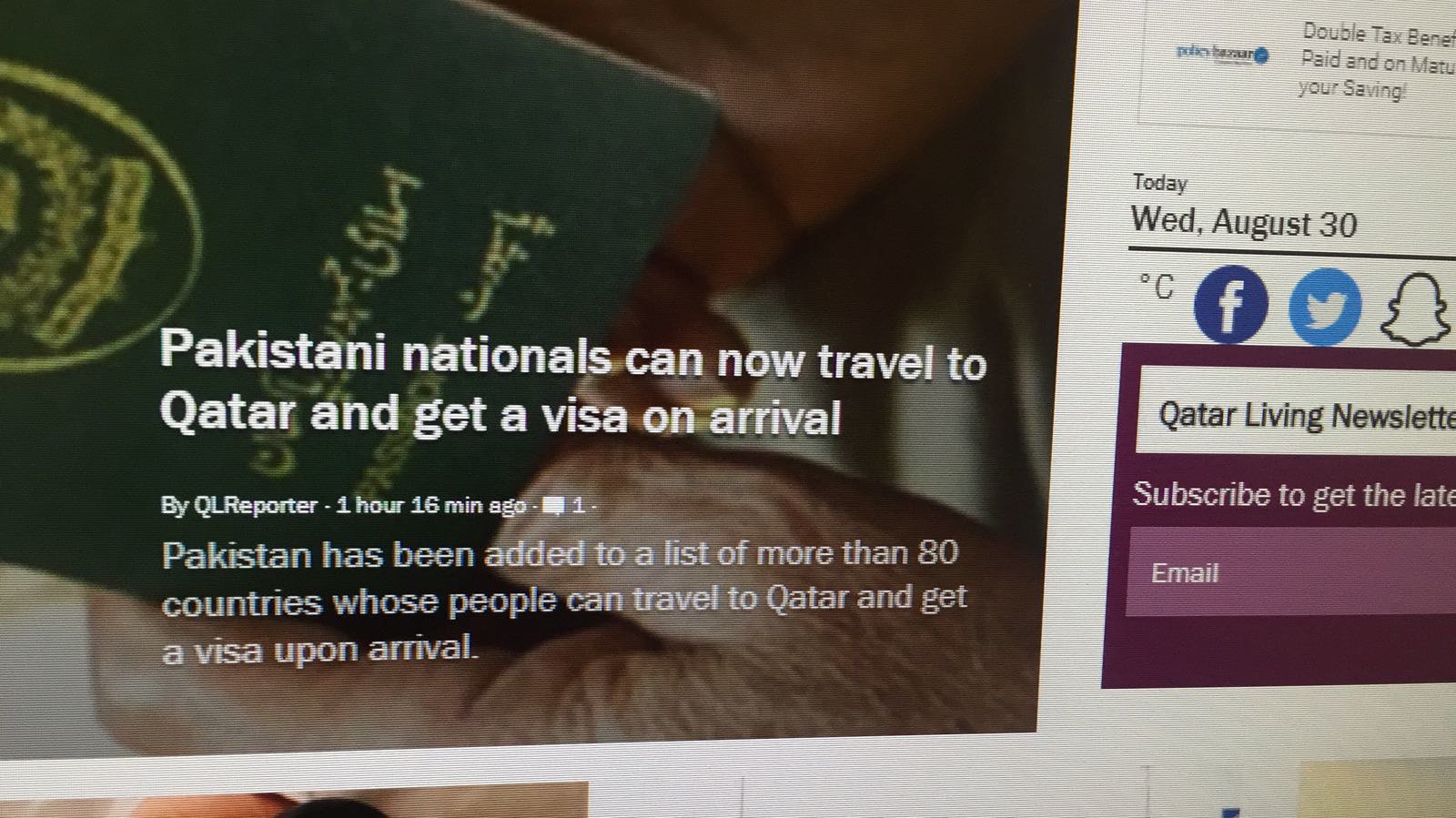The image is a detailed screenshot of a website, with a solid white background and various interactable elements. Dominating the left two-thirds of the screen is an article featuring a close-up photograph of a person holding a green Pakistani passport with gold lettering. Superimposed on the photo is large white text stating, "Pakistani nationals can now travel to Qatar and get a visa on arrival." Below this headline, in smaller white text, it reads, "By QLR Reporter, one hour 16 minutes ago. Pakistan has been added to a list of more than 80 countries whose people can travel to Qatar and get a visa upon arrival."

On the right one-fourth of the screen, a column contains additional website elements. At the top, partial text starting with "double tax benef..." is visible but cut off. Below it, the screen displays, "paid and on matu..." which is also incomplete. Further down, it reads, "You're saving," followed by the current date, "Wednesday, August 30th," and a weather indicator showing degrees Celsius without specific temperature. Social media icons for Facebook, Twitter, and Instagram are also displayed.

Beneath these icons is a maroon box with a white rectangle outlining the text "Qatar Living Newsletter." It prompts viewers to "subscribe to get the latest," followed by a field to input an email address.